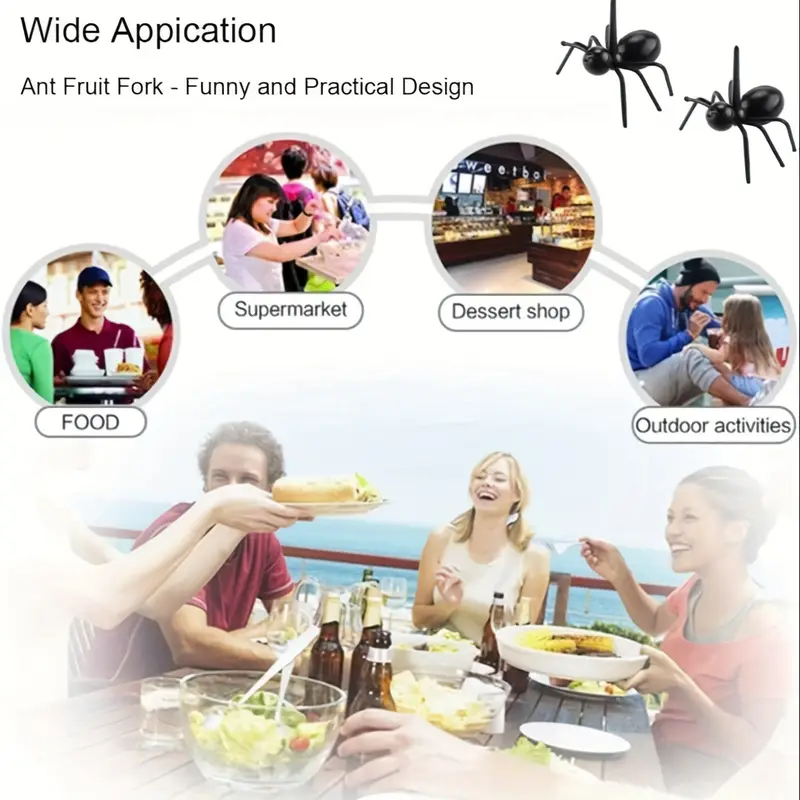This vertical rectangular advertisement features the "Ant Fruit Fork," highlighting its wide application and boasting a funny and practical design despite the slight misspelling of "application" in the tagline. In the upper left, the black text markets its versatility: "wide application – Ant Fruit Fork – funny and practical design." The upper right corner showcases two plastic ants with six legs, resembling spiders due to their round bodies and heads, complete with a large spike protruding from their backs. Below these ants, four circular photographs form an arc, depicting various application scenes like food preparation, supermarkets, dessert shops, and outdoor activities. Each scene illustrates people enjoying food and beverages, sharing laughter and camaraderie, although notably, no one is using the product. The bottom section portrays people seated around a table, happily engaged in a meal by the water, further emphasizing the fork's intended, albeit poorly demonstrated, use in social dining settings.